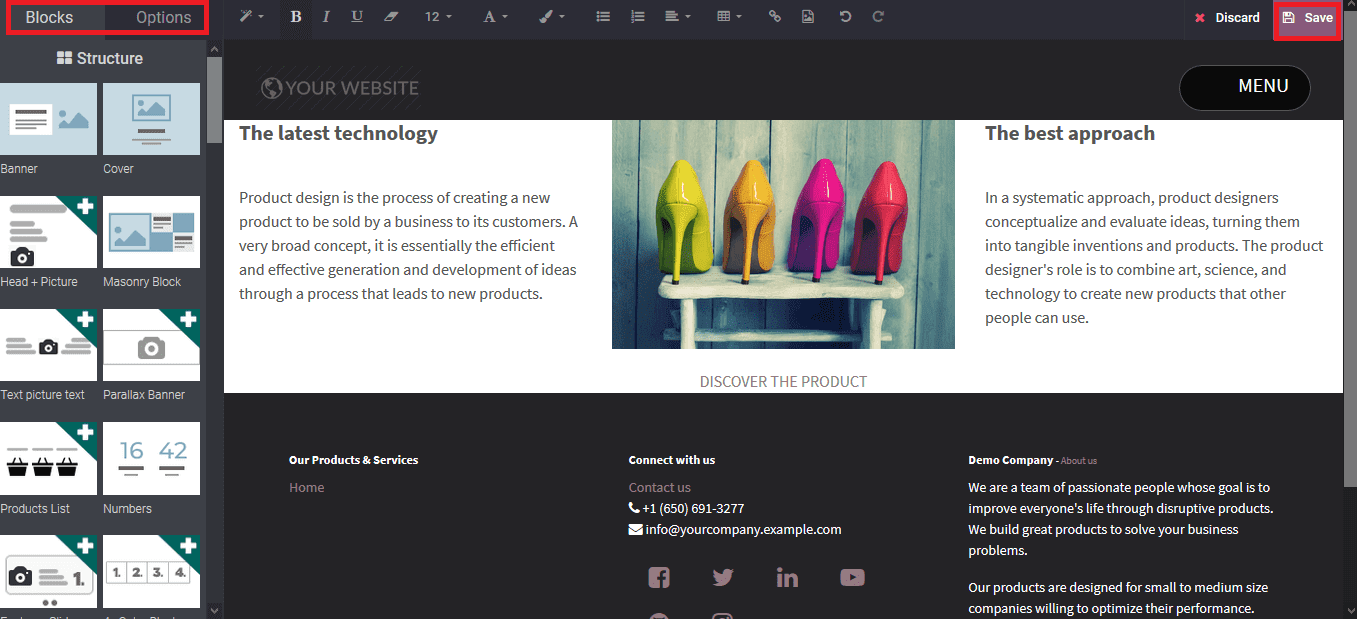This image is a cropped desktop screenshot showcasing either a website or a software tool designed for web design. The interface is not fully visible, making precise identification challenging. 

At the top of the screenshot, a menu section titled "Blocks and Options" is prominently highlighted in red, indicating it's providing instructional guidance. Adjacent to this is a comprehensive formatting toolbar featuring various icons and functions: an unclear icon, bold, italics, underline, an eraser tool, font size, font style, font color, bulleted list, numbered list, text alignment options, and a grid format. Additional icons include a phone symbol, an image insertion tool, go back and forward arrows, a red X for discard, and a red-highlighted floppy disk for saving progress.

Beneath the "Blocks and Options" menu are selectable structural elements for web design. Options such as banner, cover, head-in picture, masonry block, text-picture-text, parallax banner, product list, and numbers are visible, with more options presumably available off-screen.

Amid the workspace, a section titled "Your Website and Menu" is observed, featuring an image of vibrant high-heeled shoes displayed on a small table. The shoes are colored in neon green, mustard yellow, bright hot pink, and fire engine red. Accompanying this image, text to the left reads, "The latest technology: Product design is the process of creating a new product to be sold by a business to its customers. A very broad concept, essentially the efficient and effective generation and development of ideas through a process that leads to new products." Directly beneath the image, the caption "Discover the Product" is written, while to the right, it states, "The Best Approach: In a systematic approach, product designers conceptualize and evaluate ideas, turning them into tangible inventions and products. The product designer's role is to combine art, science, and technology to create new products that other people can use."

Towards the bottom of the screenshot, there's a navigation bar listing sections like "Our Products and Services," "Home," "Connect with Us," and "Contact Us," with contact details provided — "1-650-691-3277" and "info@yourcompany.example.com." Social media icons for platforms including Facebook, Twitter (pre-X), LinkedIn, and YouTube are partly visible.

On the bottom right, a footer section labeled "Demo Company" presents an "About Us" blurb: "We are a team of passionate people whose goal is to improve everyone's life through disruptive products. We build great products to solve your business problems. Our products are designed for small to medium companies willing to optimize their performance."

Overall, this screenshot appears to depict a web design software tool, offering various features for website construction and content organization.